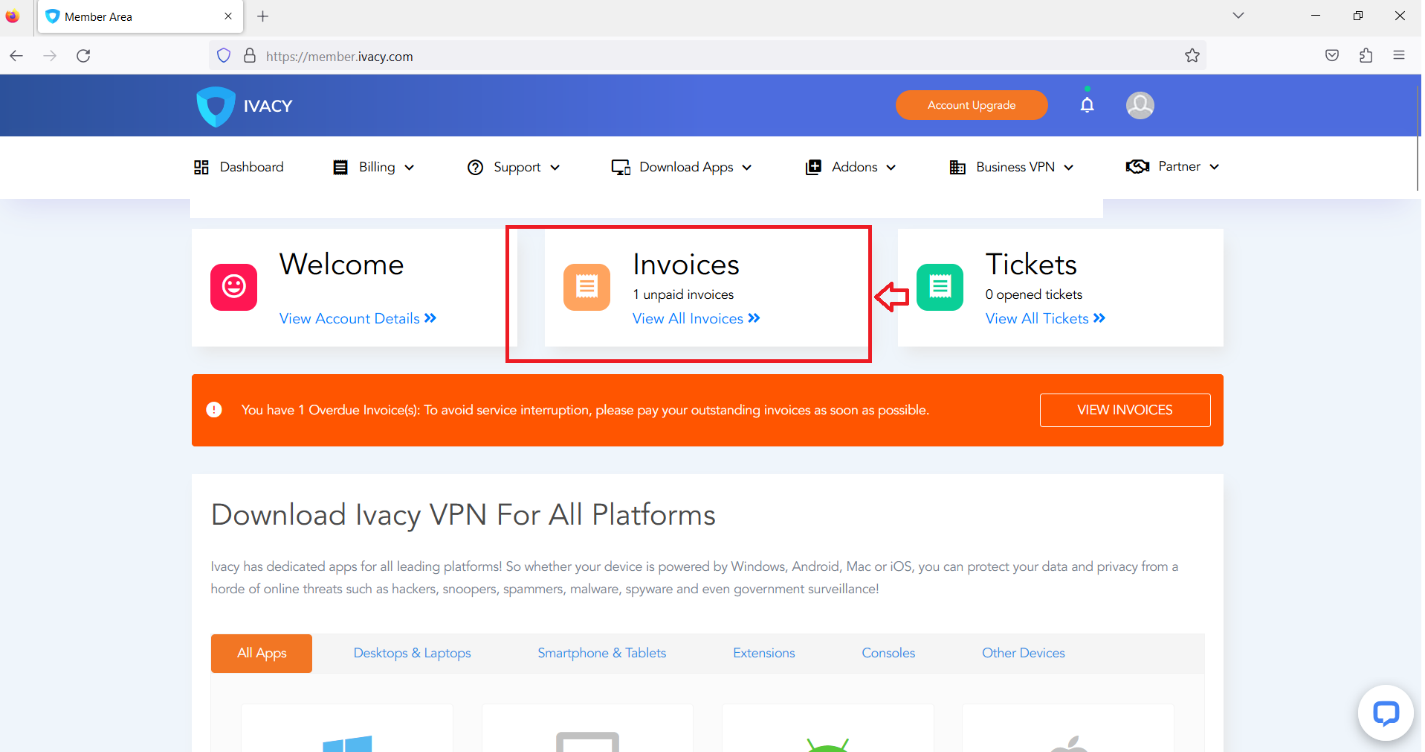This image showcases the user interface of the IVACY website's member area. At the very top, the site features a distinctive blue border, within which "IVACY" is prominently displayed in white text. An orange bubble adjacent to the IVACY logo invites users to "Account Upgrade." The navigation bar directly below this includes several tabs: Dashboard, Billing, Support, Download Apps, Business VPN, and Partner. There's an additional unreadable tab.

The central section of the page is dominated by a red-outlined box containing critical user account information. In black text, it highlights "Invoices" and notes that there is "1 unpaid invoice." A blue link below this section, accompanied by a right-facing arrow, allows users to "View All Invoices." Next to this, there is a white rectangular box labeled "Tickets," stating "0 open tickets." Similarly, a blue link with a right-facing arrow beneath this provides access to view all tickets. A red arrow points left towards the "Invoices" box.

Beneath these sections, an orange-bordered warning area features a white circle with an exclamation mark. It informs the user that they have one overdue invoice and advises prompt payment to avoid service interruption. A clickable box labeled "View Invoices" is located just below the warning message.

Further down, the page promotes downloading Ivacy VPN for all platforms. It includes multiple tabs in an orange rectangular section labeled "All Apps" with categories for Desktops and Laptops, Smartphones and Tablets, Extensions, and Other Devices. There is an additional unreadable tab in this section as well.

Overall, the detailed layout guides users through account management and service continuation, ensuring that critical information and action items are clearly visible.